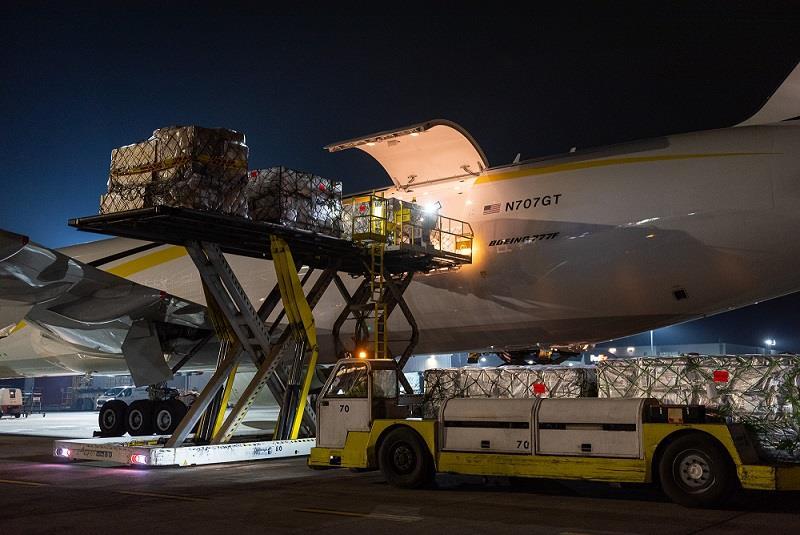The photograph captures a nighttime scene at an airport where a Boeing 777F aircraft, adorned with an American flag beside its identification number, stands stationary with its side cargo door open. The plane's sleek white body features distinctive blue and yellow stripes running along its length. Visible in the frame is a large, yellow and white service vehicle resembling a fire engine, marked with the number 70 on its side. This vehicle is equipped with a scissor lift, which is hoisting a platform loaded with secure packages wrapped in nets or plastic up to the aircraft's cargo bay. There are no humans visible in the image, suggesting that they are either out of frame or inside the aircraft, diligently working to load or unload the goods in preparation for or just arriving from flight.